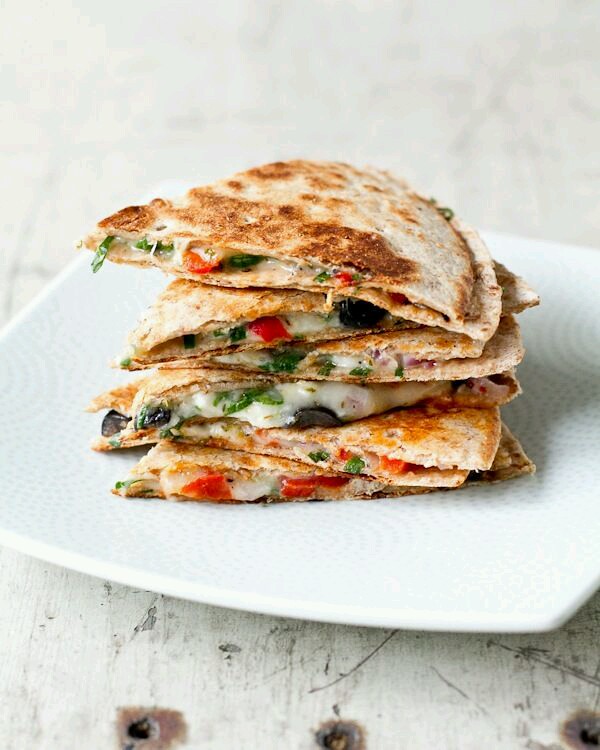The photograph depicts a square white porcelain plate with light blue circular patterns, placed on a partially aged white wooden table marked by black lines and browned nail holes. On the plate are six golden-brown, crispy pieces of bread or paninis, generously filled with a mix of melted cheese, green asparagus, and red bell peppers, as well as some black olives. The savory filling oozes out from the lightly crusted edges of the grilled bread, offering a colorful contrast of white, red, green, and black hues.